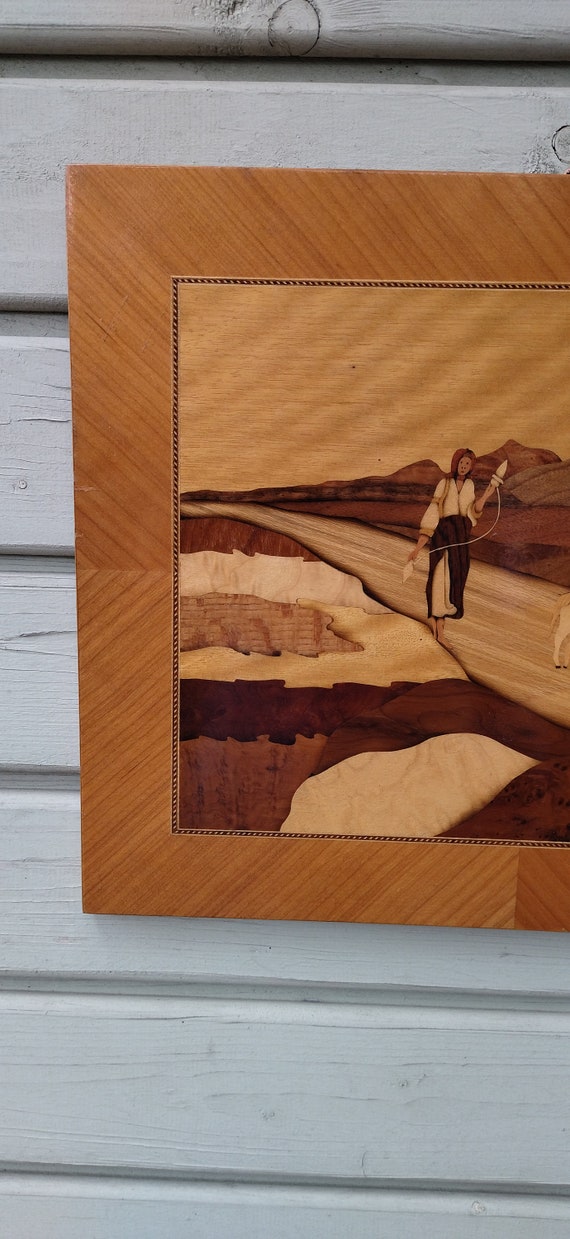The image showcases a framed painting hanging on a wall constructed of horizontal wooden beams painted in a light, almost white, gray. The wooden frame of the painting features distinct wood grains and is brown in color, blending harmoniously with the neutral tones of the painting it holds. The scene within the painting depicts a vast, open road flanked by a rugged terrain of canyons, mountains, and a field, all painted in earthy shades of brown, white, and a hint of mahogany. The painting's dominant colors are neutral, creating a serene Western ambiance.

At the center of the painting stands a solitary figure, possibly a cowboy or an archer, dressed in brown and white, holding either a bow or perhaps a rope or kite; the details are indistinct. The sky above is a striking orangish brown, enhancing the overall Western theme that seems to celebrate the rugged, agrarian ideal of the West. There are no textual elements in the image, allowing the viewer to fully immerse in the evocative, desolate beauty of the scene. The painting is partially cut off in the photograph, positioned towards the middle to the right of the composition, and is devoid of any additional written context.